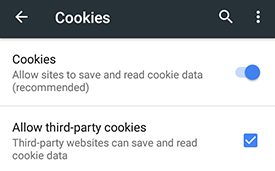A screenshot of a cookies management interface, possibly from a web browser or an application. The top section features a black navigation bar. On the far left of this bar is a left-pointing arrow icon, followed by the label "Cookies" in white text. To the right of the bar are a search icon (magnifying glass) and a vertical ellipsis (three dots arranged vertically).

Below the navigation bar is the cookies management content. The first section on the left is titled "Cookies" with the description: "Allow sites to save and read cookie data (recommended)." Below it is another option labeled "Allow third-party cookies," accompanied by the description: "Third-party websites can save and read cookie data." Both cookie options are toggled on, indicating that the site or application permits storing and reading cookies by default.